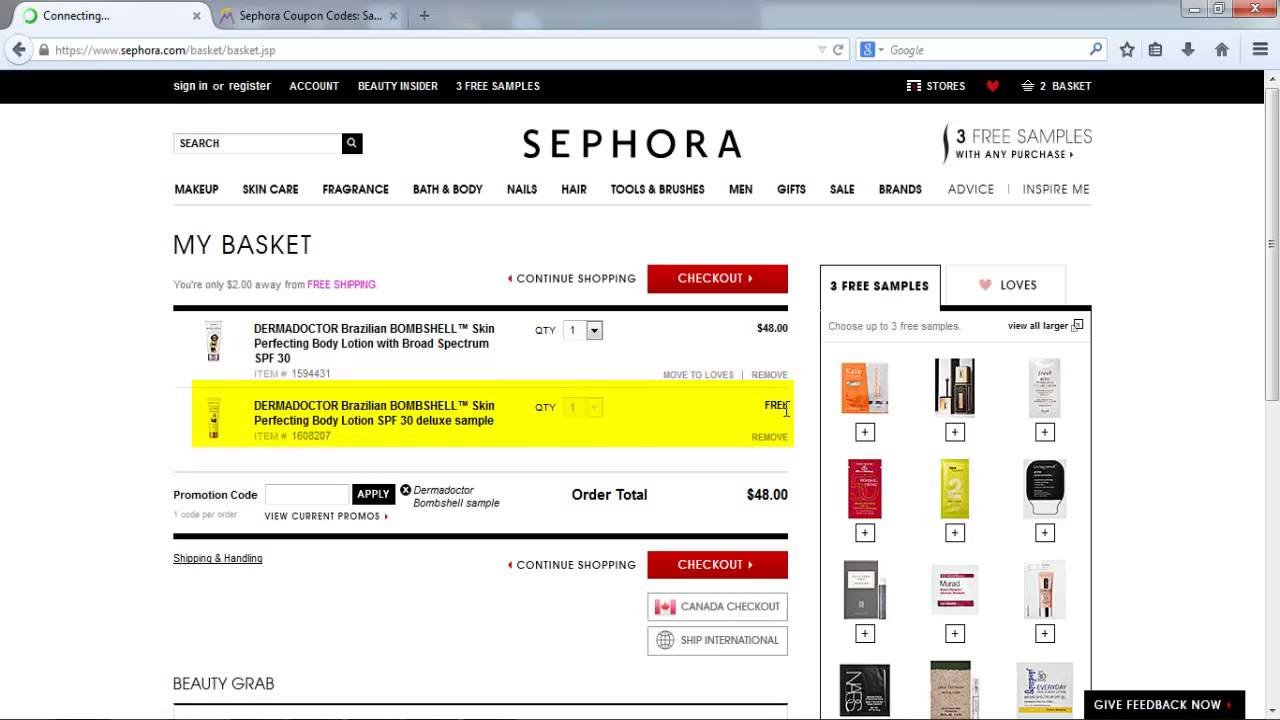This is a detailed screenshot of a website browser displaying the Sephora homepage. The page features a white background and a prominent black header. On the left side of the header, there is indented white text in lowercase that reads "sign in or register." To its right, separated by a small space, there's white text in all caps that lists: "account," "beauty insider," and "3 free samples." Following a large area of negative space to the right, there is a white icon consisting of three horizontal bars stacked vertically, adjacent to another similar icon, both bridged by a longer horizontal bar.

Next, moving rightwards, the header continues with white text in all caps that reads "stores," followed by a red heart icon, a white shopping basket icon, a white numeral "2," and lastly, more white text in all caps that says "basket."

In the main body of the page, centrally at the top, there is large black, all caps sans-serif text that states "SEPHORA." To the left of this, after some negative space, is a white search bar outlined in medium gray. The search bar contains black, all caps text on the left that reads "search," and on the right side, there is a black square with a white magnifying glass icon inside it.

To the right of "SEPHORA," past some negative space, appears a black shallow S-curve. This is followed by two lines of text: the first line, in larger font, consists of a black numeral "3" and light gray, all caps text that says "free samples." The second, smaller line underneath displays black, all caps text that reads "with any purchase." To the right of this text, there is a black arrow pointing to the right.